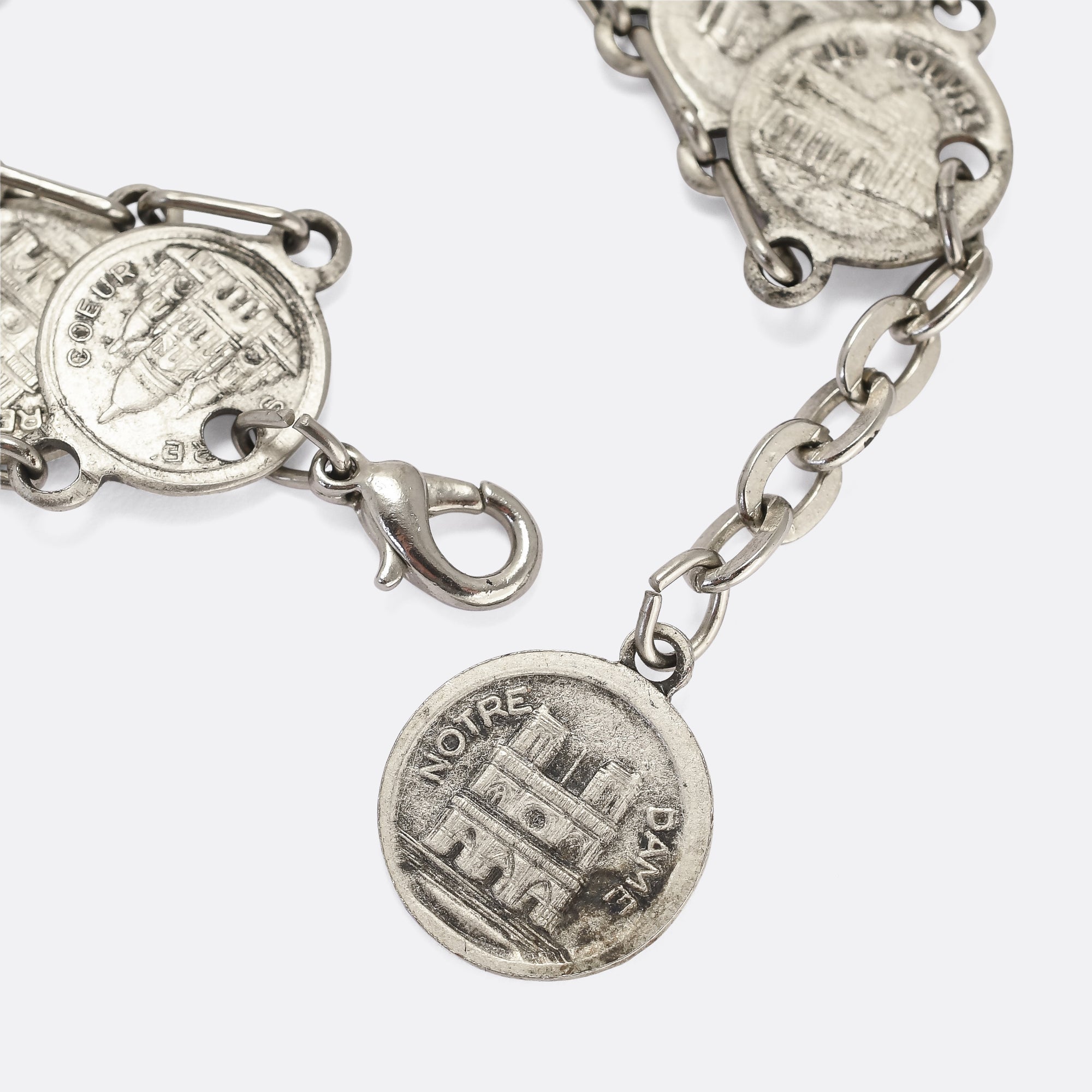The image depicts a piece of silver jewelry against a white background, likely a necklace or bracelet, featuring several coin-shaped medallions attached to a thin chain. At the top of the picture, one of the coins, which is slightly larger, bears the inscription "Le Louvre," referencing the famous Parisian museum, with an indented representation of the structure. Further down the chain, in the middle of the image, another medallion is engraved with "Notre Dame" and features a depiction of the iconic cathedral. To the left of the "Notre Dame" coin, another medallion is connected to the chain, inscribed with "Cœur," and showcases an image of the Sacred Heart basilica. The chain features various thick silver links and ends with a standard jewelry clasp mechanism, which can be pressed down to open. The metal of the medallions and chain appears to have a slightly tarnished, gritty texture, adding a touch of antiquity to the piece.